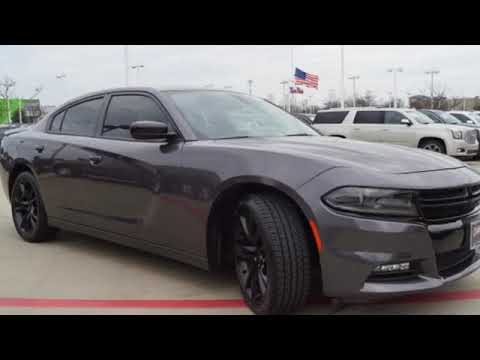The photograph features a dark gray Dodge Charger positioned at a 45-degree angle with the passenger side prominently displayed. The car's front end faces the right front corner of the image, with the front wheel turned towards the background, suggesting the vehicle is turning. The Charger boasts tinted windows and lights that are off. The scene appears to be set in a parking lot, possibly at a car dealership, as indicated by the street lights on white poles. In the background, a row of parked vehicles, including a large white SUV likely a Cadillac Escalade, is visible. An American flag is floating above the cars, and a bright green building can be seen in the top left corner. The ground is a tan-colored pavement with a red stripe running horizontally in front of the Charger. The photograph has a thin black border at the top and bottom.